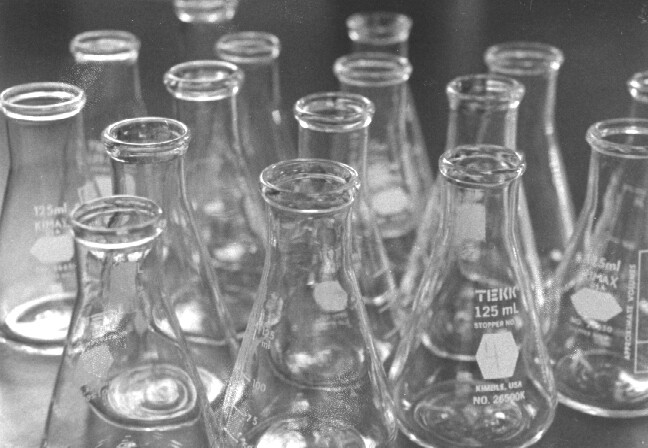This black and white photograph features an array of clear glass flasks, each with a canonical shape characterized by a narrow neck that widens toward the base. Spanning approximately four visible rows, the flasks are meticulously arranged on what appears to be a metal or gray surface, with a similarly hued background. The forefront of the image prominently displays three flasks, among what looks to be a total of 15 to 20. Each flask is marked with white lettering that reads "TEKK, 125 mL" alongside a white octagonal (or hexagonal) emblem and what seems to be a patent number, indicative of their high-quality and sterile condition, making them ready for immediate laboratory use. The flasks are roughly six inches tall and are devoid of lids, suggesting they are prepared for various scientific experiments involving liquid handling. The image captures the flasks in neat, horizontal alignment, presenting a clean and orderly display, whether for use or observational purposes.